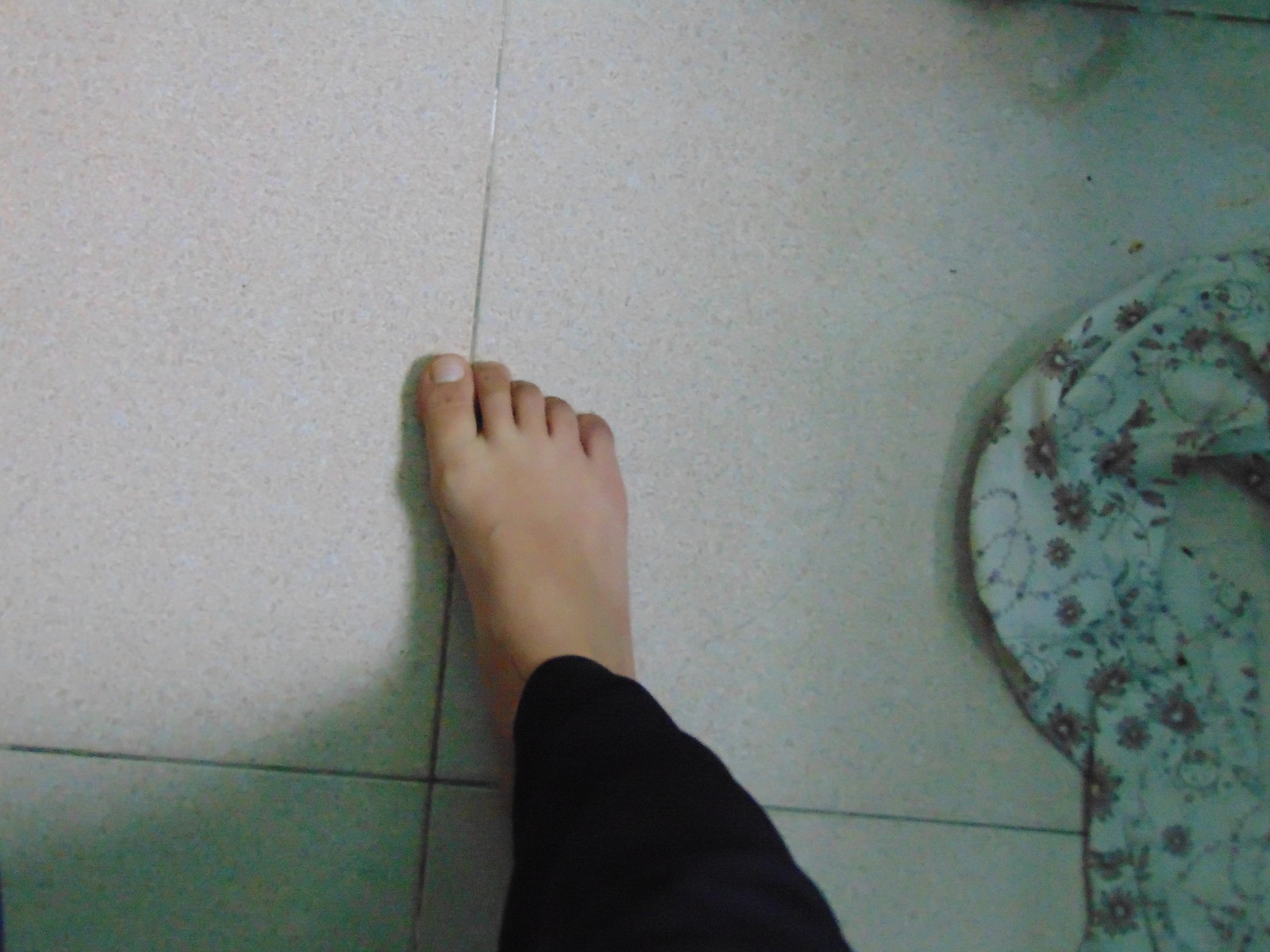This image features a close-up of a person's right leg and foot, positioned on a tiled floor with thin gray grout lines. The individual, who appears to be female, is barefoot and wearing black sweatpants that extend down to the ankle. The photograph is taken in what seems to be a bathroom, suggested by the items and clothes scattered off to the right side, including a white fabric with a pink floral pattern and looping vines. Additionally, a stain is visible on one of the white tiles in the top right corner of the image.